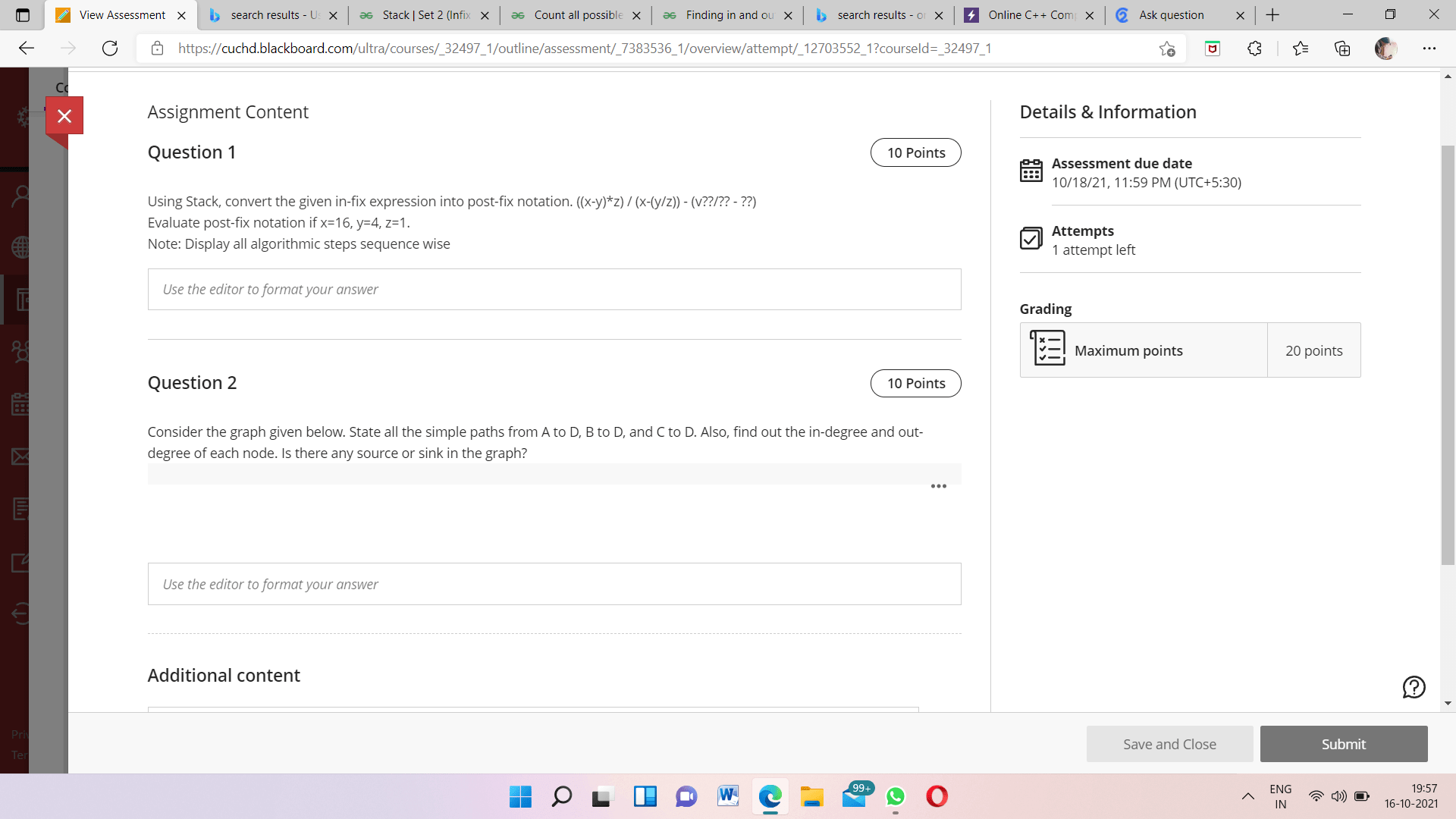This is a detailed screenshot taken from a web browser, specifically Microsoft Edge. The top section of the browser shows 8 open tabs arranged from left to right as follows: "View Assessment," "Bing Search Results," "Stack Set To," "Court of All Possibilities," "Fencing In and Out," another "Bing Search Results," "Online C++ CO," and "Ask Jeeves."

The primary focus of the screenshot is on the first tab labeled "View Assessment." The webpage displayed has a clean white background with a header that reads "Assignment Content." Under the header is "Question 1," which instructs users to convert a given infix expression into postfix notation using a stack. The exact mathematical formula is too small to discern clearly in the screenshot. Additionally, the assignment requires evaluating the postfix notation given the values x = 16, y = 4, and z = 1. The task also specifies that all algorithmic steps should be displayed sequentially, and it is valued at 10 points.